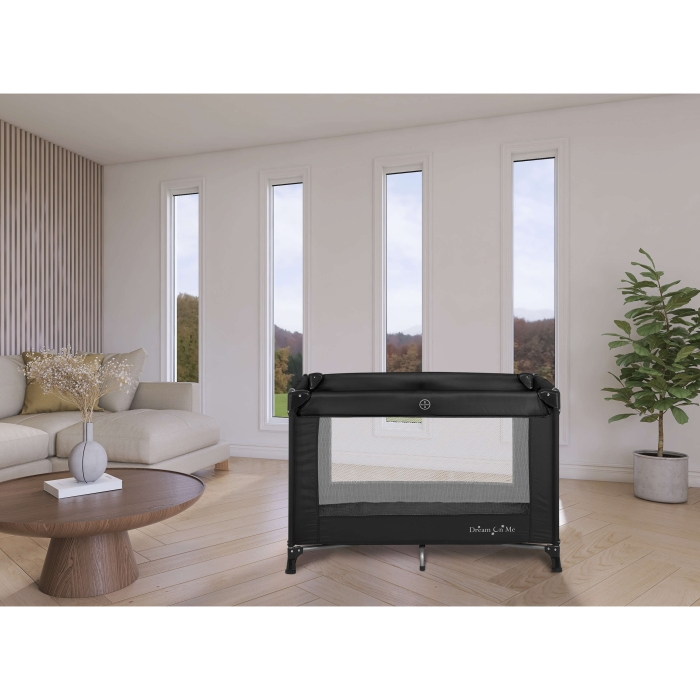A modernistic living room bathed in natural light streams in through four tall, slender vertical windows on the back wall. The room features a brown wooden floor and is decorated with a mix of contemporary furniture and natural elements. Dominating the left side is a sleek white couch, beside which stands a wooden coffee table that supports a small vase filled with brown flowers. On the right, a potted plant resembling a small tree brings a touch of greenery to the space. Central in the room is a black playpen with mesh sides and six legs, elevated slightly off the floor. The playpen, positioned towards the bottom right of the image, has a logo reading "Dream On Me" in white letters on its lower right corner. The windows provide a view of lush hills filled with trees, contrasting beautifully with the room's modern aesthetic.